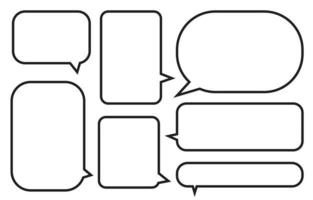The image features a collection of seven distinct speech bubbles, commonly found in comics, displayed against a solid white background. These dialogue boxes, outlined in black with white interiors, vary in shape and size, creating a dynamic grid-like arrangement. In the upper left is a horizontally-oriented square bubble, followed by a slightly rounded vertical rectangle and an oval-shaped bubble in the top right. The middle section showcases two vertical square-like bubbles. Below, there's a larger, more rectangular bubble with soft corners, flanked by another long rectangular one, and a long oval bubble. Each speech bubble's directional pointer varies, aiming downwards, to the left, and to the right, but none upwards. This intricate assortment is meticulously organized, highlighting the diversity of forms that speech bubbles can take in visual storytelling.